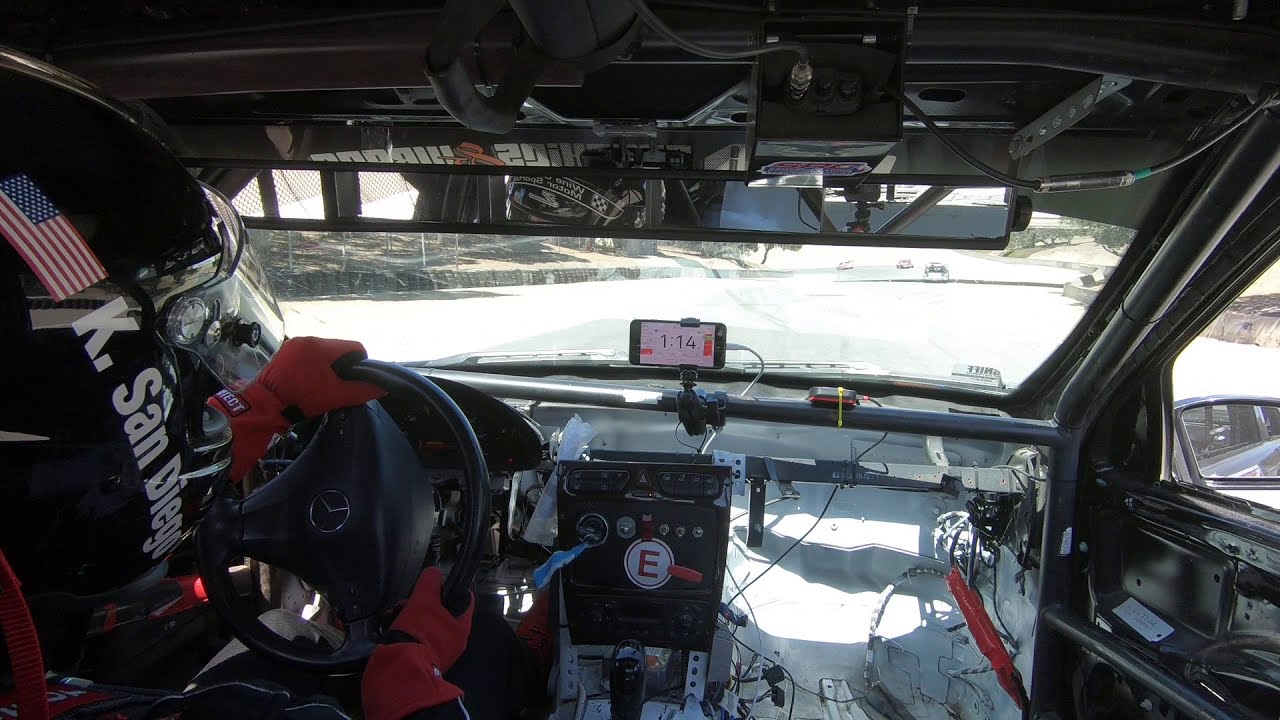This photograph captures the interior view of a racing car from a vantage point behind the driver, who is positioned on the left side of the image. The driver is adorned in red gloves and a black helmet, prominently featuring an American flag and the text "K. Santiago." The driver's hands grasp a black steering wheel amidst a dashboard cluttered with wires and essential racing instruments. A phone displaying the time "1:14" is mounted at the center of the dashboard. Visible through the windshield is a bright, white racetrack with a few other sports cars ahead in the distance, underscoring the competitive racing environment.